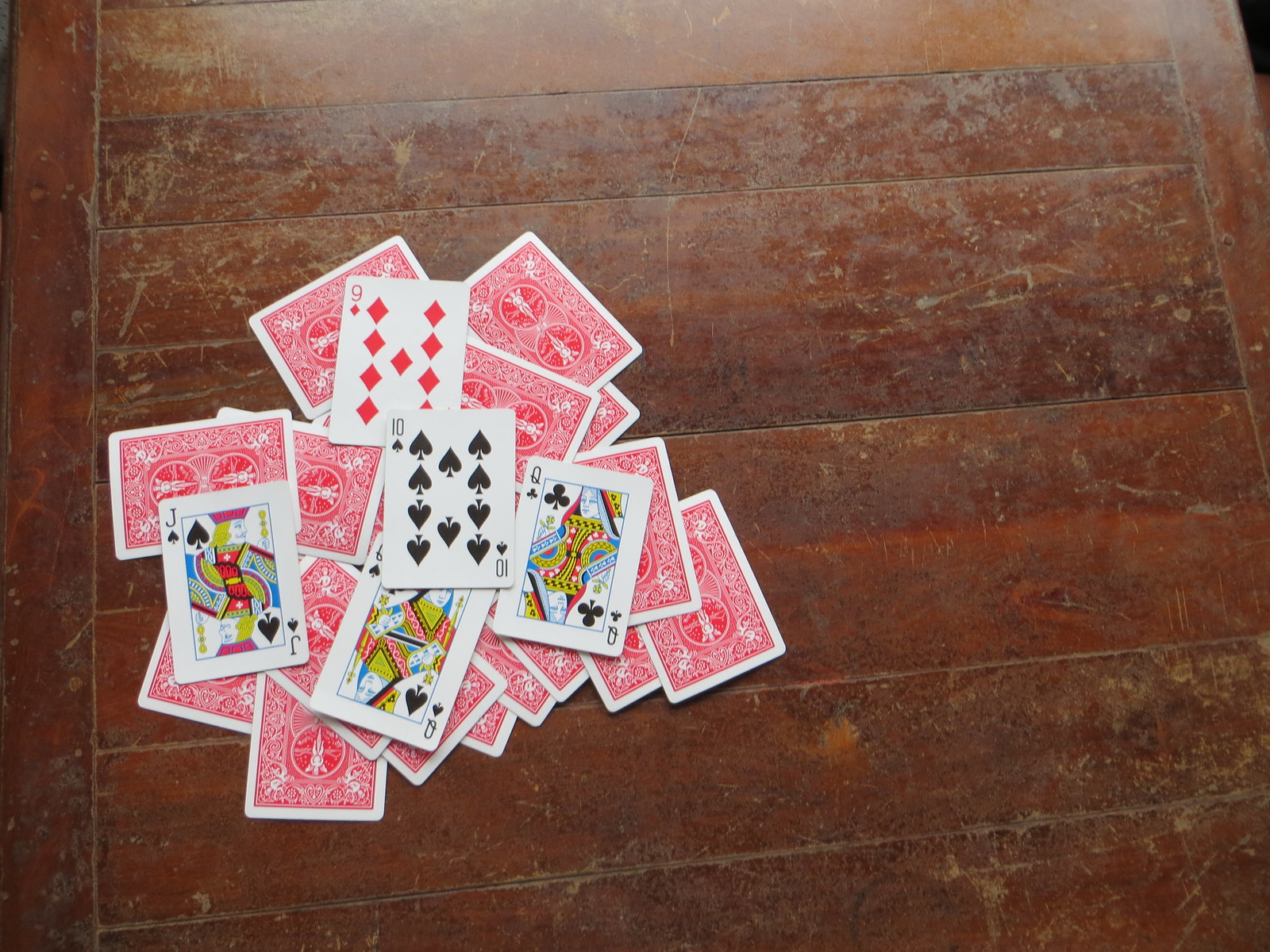This image features a well-worn table, its surface marred by numerous scratches and dings, revealing the passage of time. The table's original medium brown hue, once interspersed with subtle dark striations, is now heavily faded and discolored, especially on the top where the finish has been significantly rubbed away. At the focal point of the scene, a haphazard pile of playing cards rests on the table. The majority of the cards lie face down, their values hidden, but five cards are visible: the jack of spades, the queen of spades, the queen of clubs, the ten of spades, and the nine of diamonds. The random assortment of cards contrasts starkly with the table's well-worn surface, hinting at many games played and stories told.